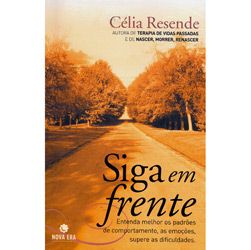This book cover, likely in Spanish, presents an evocative scene of a road flanked by two rows of trees—yellow and orange-hued on the left, and white-trunked trees on the right—leading into the distance. Dominated by an orangey shade, the cover features the author's name, Celia Resende, in red font at the upper right corner. Below the author’s name, there are some smaller, unreadable words. The title, "Siga em Frente," appears towards the bottom right, italicized, and perhaps followed by a brief summary, also too small to decipher. The overall image captures a serene, distant perspective of the path amid an autumnal setting.